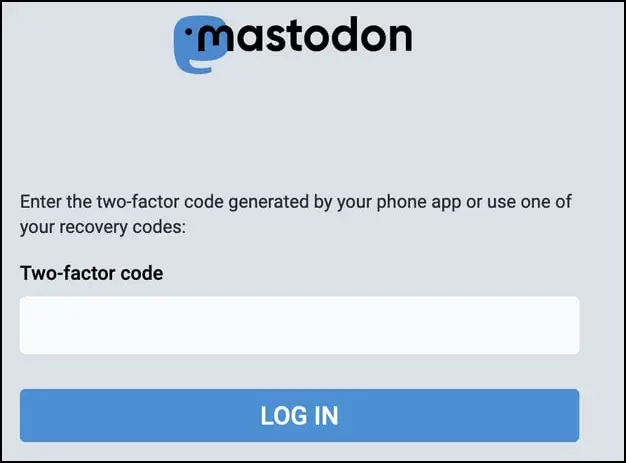The image depicts a login interface for a website, specifically Mastodon. The interface is framed within a gray square outlined in black. Within the gray frame, there is an illustration of a whale near the letter 'M' in the Mastodon logo, both in lowercase black lettering. Below the logo, text prompts the user to enter their two-factor authentication code generated by a phone app or to use one of their recovery codes. 

The instructions read: "Enter the two-factor code generated by your phone app or use one of your recovery codes." Following this, an additional line states: "I don't need that:" followed by a prompt for the two-factor code.

Underneath these instructions, there is a white rectangular input box that spans from left to right, designed for users to enter their two-factor authentication code. Below this input box, there is a blue rectangular button, also extending from left to right, with the word "Login" in white text. 

Overall, the interface is neatly designed, with clear and contrasting elements to guide the user through the authentication process.